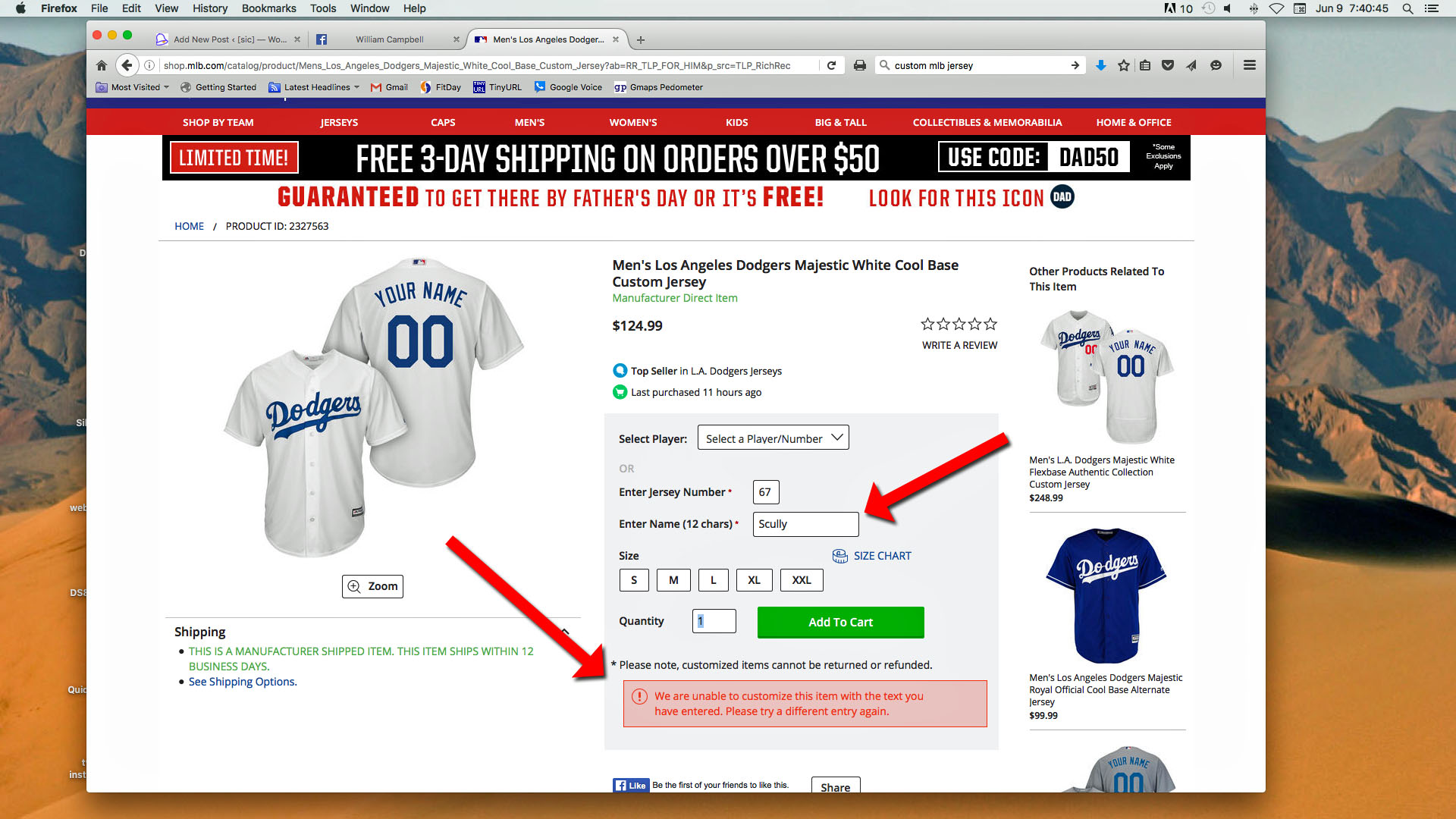A Mac OS computer is prominently displayed, featuring the default desktop background of a picturesque mountain range and sand dunes. The screen is dominated by an open web browser, most likely Chrome, although its appearance has been modified by the Mac OS interface. Three tabs are visible, with the active one focused on a Los Angeles Dodgers baseball page. The user appears to be customizing a men's Majestic White Cool Base Dodgers jersey. Several fields are available for customization, including a text box for entering a name, limited to 12 characters. The user has input "Scully," in reference to Vin Scully. Despite completing other fields, an error message at the bottom of the page reads: "We are unable to customize this item with the text you have entered. Please enter a different entry," indicating that the name "Scully" cannot be used.